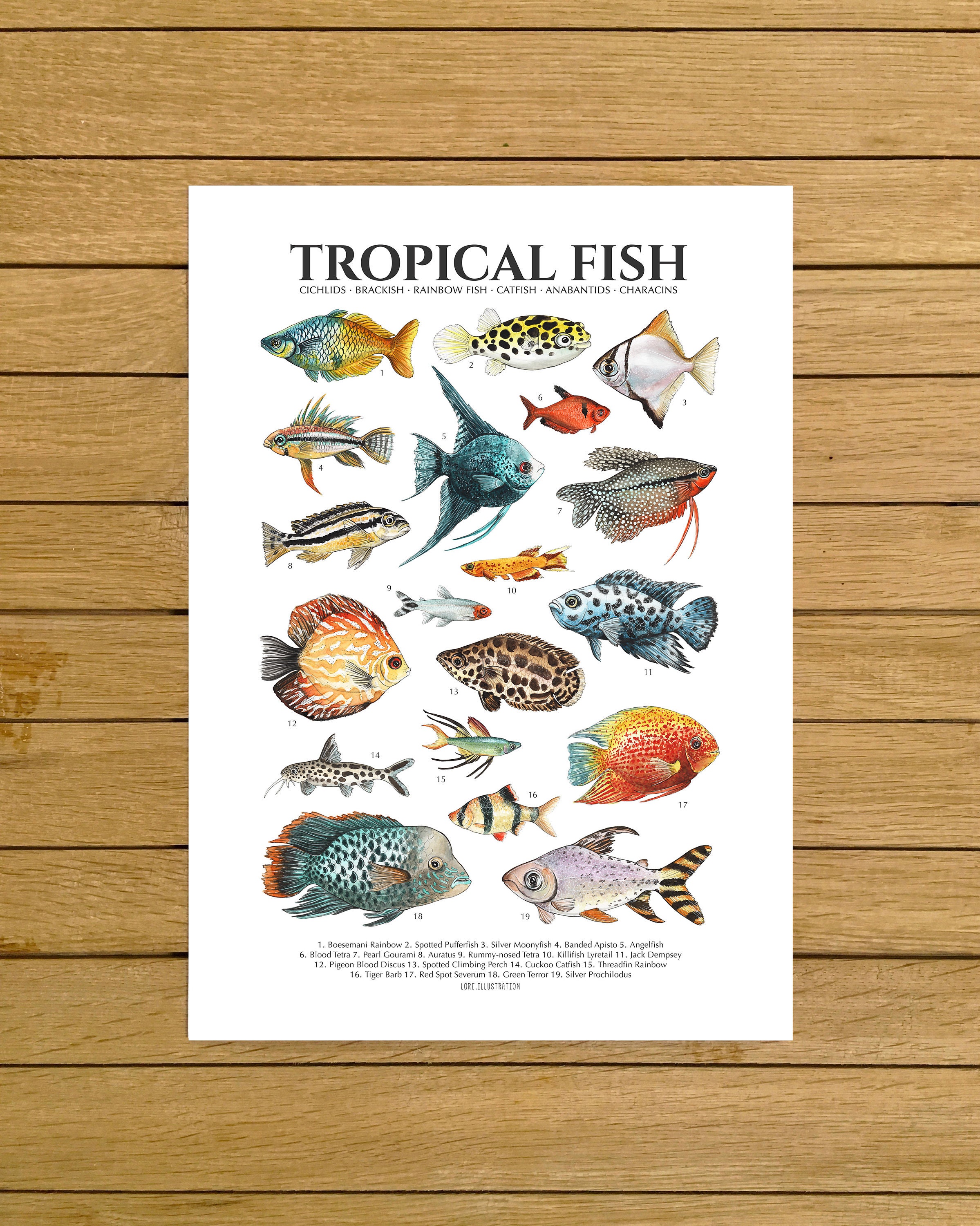This color photograph captures a white poster titled "Tropical Fish," positioned on a surface of horizontal wooden planks with distinct wood grain. The title "Tropical Fish" is prominently displayed in large black font at the top of the poster, beneath which is a smaller subheading listing various fish categories like cichlids, brackish, rainbow fish, catfish, and anabintids, though the exact text is difficult to discern. 

The main portion of the poster, approximately 80%, features colorful illustrations of around 19 different tropical fish, each uniquely depicted in a vivid palette of blues, oranges, reds, whites, greens, and blacks, highlighting their diverse shapes and patterns. Each fish is marked with a small number, and the corresponding legend at the very bottom of the poster provides the scientific names and details for each numbered fish, although this text is too tiny to read clearly.

Overall, the poster serves as a detailed, indexed guide to various tropical fish species, beautifully illustrated and systematically organized for easy identification.